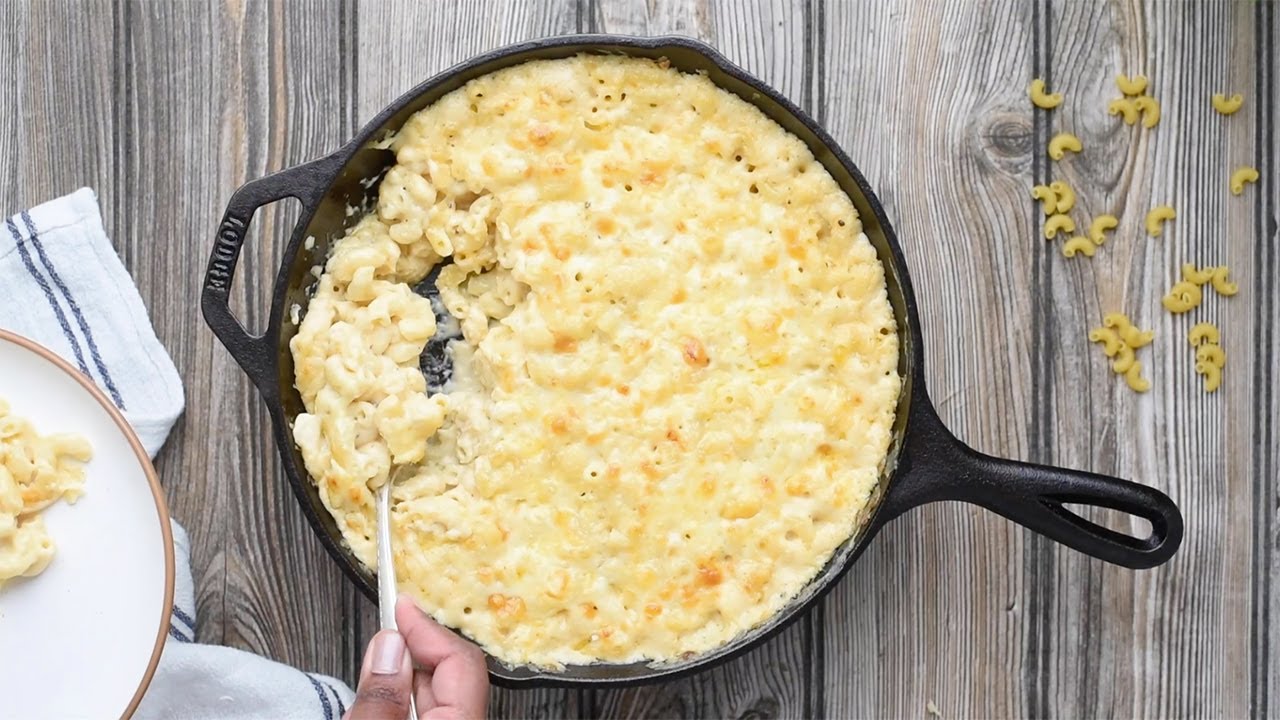The image showcases a large, black cast iron skillet filled with creamy, light orange and yellow macaroni and cheese, presumably baked in the oven. The skillet is positioned on a grayish-brown, wood-grained tabletop. To the right of the skillet, there are some scattered dried macaroni noodles. A hand with dark skin is seen in the upper right section of the image, holding a spoon to scoop out a portion of the macaroni and cheese. Below the hand, a white plate with a brown rim already holds a serving of the cheesy dish. This plate rests on a white cloth with blue stripes, completing a cozy, rustic dining setup.